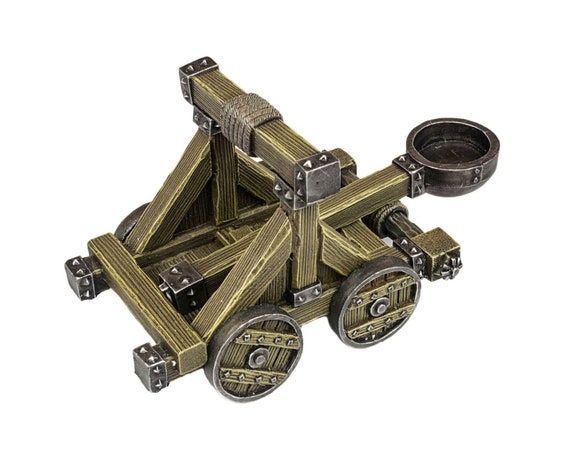This photograph features a detailed small-scale model of a medieval catapult, prominently displayed against a pure white background. The catapult is primarily constructed from square-cut timber, giving it a brown color due to the wood and rope components, while metal elements are silver. The base consists of a rectangular chassis mounted on four wooden wheels, each rimmed with metal. The central A-frame, formed by two angled beams on either side, supports the lever arm mechanism. The model's lever arm, extending to the right and equipped with a half-circle metal cup at the end, is designed to launch projectiles. The arm is propped up by two vertical posts connected by a horizontal brace at the top, with a piece of timber and rope at its center. The model includes detailed metal components, including caps with spikes and bolts that hold the structure together, enhancing its realism. The overall craftsmanship indicates it represents an 18th or 19th-century toy version of the ancient siege weapon, used traditionally to hurl rocks, boulders, or flaming coals in battle. This meticulously created model captures the essence and functionality of its historical counterpart.